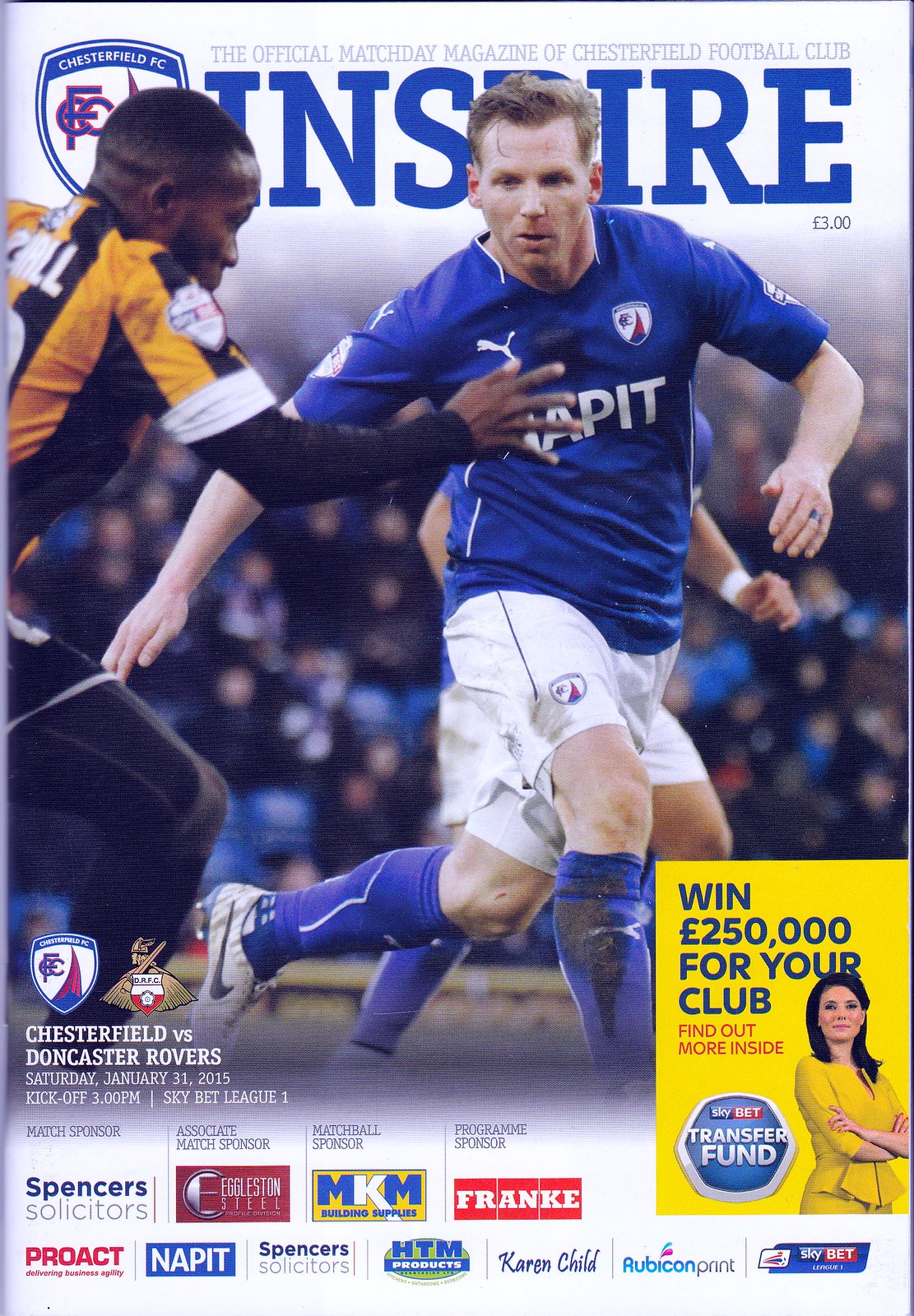This detailed descriptive caption incorporates elements from all three voice captions, with an emphasis on shared and repeated details:

"The cover of the official match day magazine of Chesterfield Football Club, titled 'Inspire,' is prominently displayed. Priced at three pounds, this magazine features a dynamic action photograph of a soccer match. To the right, a player in a blue shirt with white shorts, representing Chesterfield, is captured in mid-play. He is being challenged by an opposing player in a yellow and black striped jersey, black shorts, and leggings from Doncaster Rovers. Another player in blue is visible behind the action, further adding to the intensity of the scene. The backdrop shows a blurred crowd, creating a lively atmosphere.

At the top of the cover, the Chesterfield FC logo can be seen alongside the title 'Inspire' and the phrase 'The Official Match Day Magazine of Chesterfield Football Club.' Beneath the photo, the text announces the fixture: 'Chesterfield versus Doncaster Rovers, Saturday, January 31st, 2015. Kickoff at 3 p.m., Sky Bet League 1.' Surrounding the bottom of the cover are various sponsor logos, including Proact, NAPIT, Spencer's Solicitors, HTM Products, Karen Child, Rubicon Print, Sky Bet, Frankie, MKM, and Eggleston Steel. An advertisement on the side, featuring a woman in a yellow dress, promotes the chance to win 250,000 pounds for your club through the Sky Bet Transfer Fund, inviting readers to find out more inside."